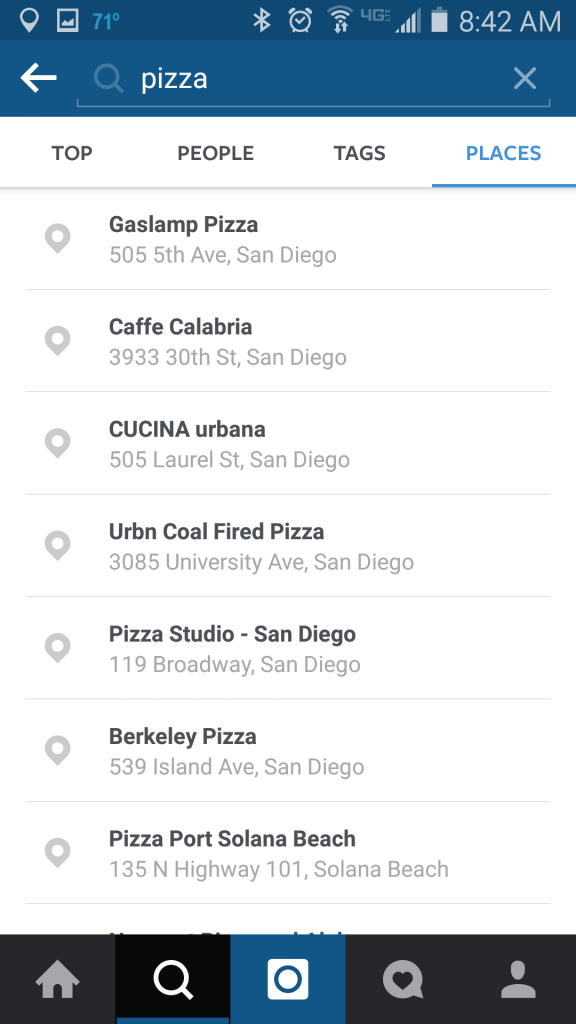In the image, an individual is seen using their smartphone to search for pizza places. The current time displayed on the phone is 8:42 a.m., and the temperature reads 71 degrees. The search query "pizza" reveals a list of results, and various app icons are visible on the screen. The top result is "Gaslamp Pizza" located at 505 Fifth Avenue, San Diego. Following this are "Cafe Calabria" at 3933 30th Street, "Cucina Urbana" at 505 Laurel Street (though there is a spelling error in the result where "Urban" is misspelled as "Urban"), "Urban Coal Fired Pizza" at 3085 University Avenue, "Pizza Studio" at 119 Broadway, and "Berkeley Pizza" at 539 Island Avenue, all in San Diego. The last listed result is "Pizza Port Solana Beach" at 135 North Highway 101, Solana Beach. The image captures the detailed search results and suggests that additional options are available for refining the search, such as underlining "places," "people," or "tags" to reclassify the results and obtain more specific information.